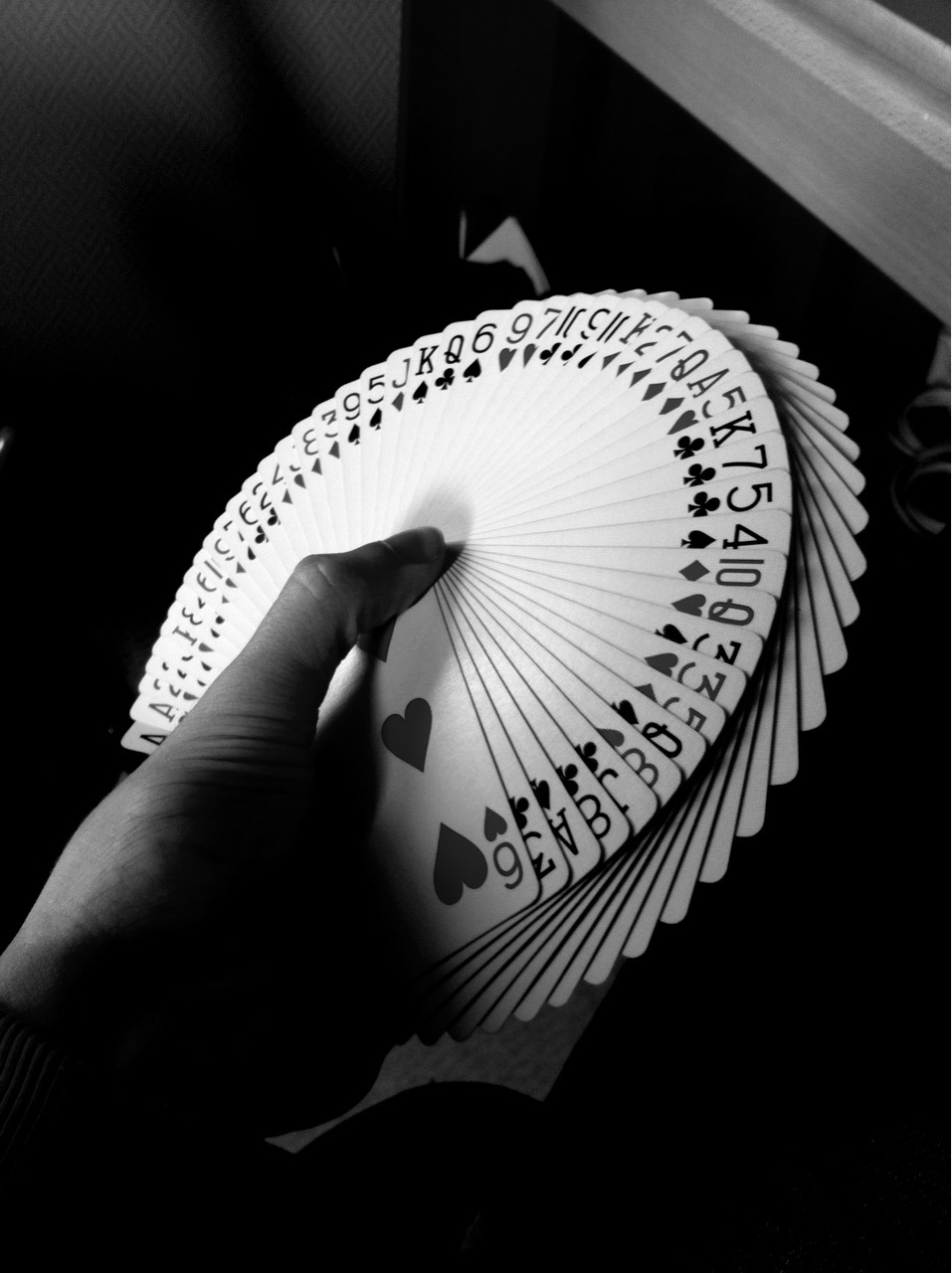This black and white photograph features a strikingly dark background, interrupted by a whitish-gray board situated at the top right corner. Emanating from the bottom left is a hand, elegantly fanned out and holding an elaborate deck of playing cards, all meticulously arranged and also in monochrome. The cards, displayed in an intricate spread, include: the six of hearts, three of clubs, ace of spades, eight of clubs, jack of clubs, eight of hearts, queen of spades, five of diamonds, three of hearts, three of spades, queen of hearts, ten of diamonds, four of spades, five of clubs, seven of clubs, king of clubs, five of hearts, ace of spades, queen of clubs, seven of hearts, two of diamonds, king of hearts, ten of hearts, nine of diamonds, six of clubs, eight of hearts, king of spades, jack of diamonds, five of spades, nine of spades, three of diamonds, eight of diamonds, four of hearts, two of spades, six of diamonds, seven of spades, nine of clubs, and ace of hearts. Some cards are partially obscured, adding an enigmatic quality to the image, but prominently showcased at the end of the spread are two aces, symbolizing a climax to the visually rich arrangement.